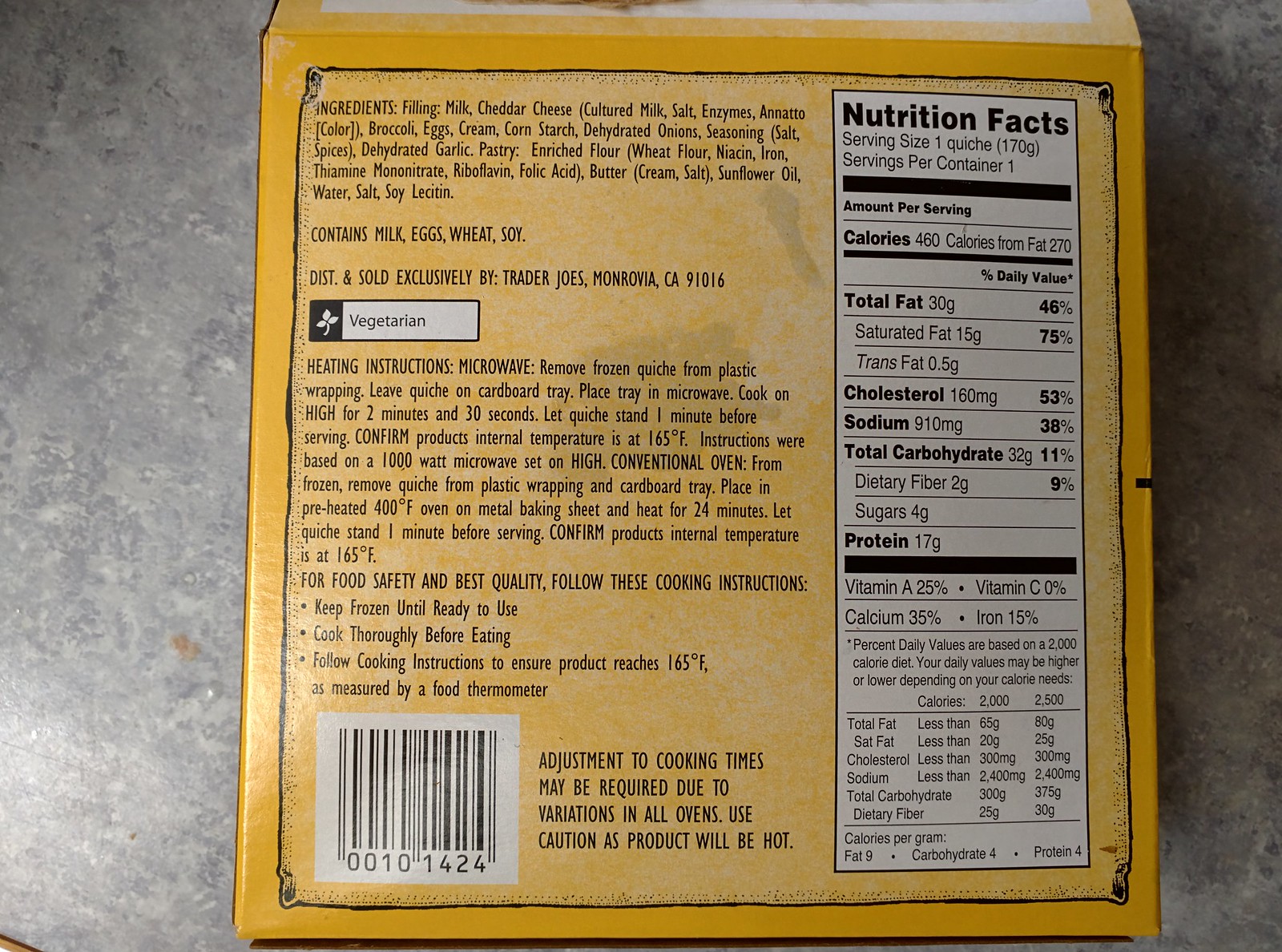This image captures the back panel of a microwavable food product package, exclusively sold at Trader Joe's. The product's box is vividly yellow, drawing attention to its detailed ingredient list. The filling consists of milk, cheddar cheese, broccoli, eggs, cream, cornstarch, dehydrated onions, seasoning, and dehydrated garlic. The pastry ingredients include enriched flour, butter, water, salt, and soy lecithin. Clearly stated, the product contains milk, eggs, wheat, and soy. This vegetarian item is distributed and sold solely by Trader Joe's, located in Monrovia, California, 91016. The bottom section of the panel features clear heating instructions for customer convenience.